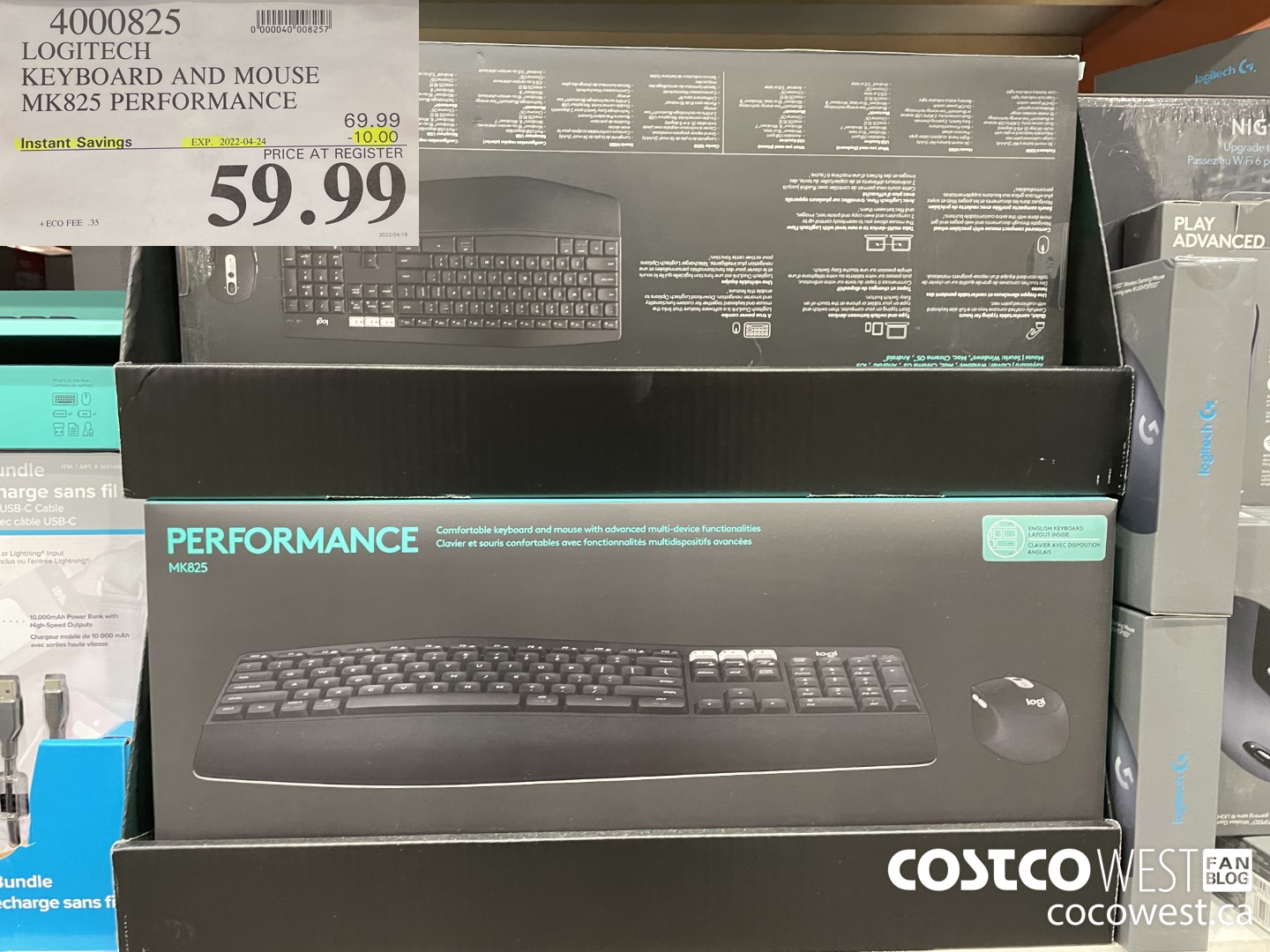This image depicts a photograph of a Logitech keyboard and mouse set, specifically the MK825 Performance model. The box, predominantly black in color, features a detailed life-size image of the black keyboard with a built-in wrist guard and mouse. Prominently displayed in the upper left corner of the box is the branding "Logitech Keyboard and Mouse, MK825 Performance." Additionally, there is a notification of an instant savings offer that expires on 2022-04-24, reducing the original price from $69.99 to $59.99 after a $10 discount at the register. 

Furthermore, the image specifies an ECO fee of $0.35, and a product number identified as 400-030-825. At the bottom, the box advertises the Costco West Fan Blog with its website, CocoWest.ca, in white font. Running across the top left side, the text "Performance" is displayed. The box also highlights the product’s key feature of being a "Comfortable Keyboard and Mouse with Advanced Multi-Device Functionalities," which is repeated in French below it, both in green font against the black background. Additionally, a circular insert provides a close-up view of the keyboard and mouse, showcasing their intricate details.